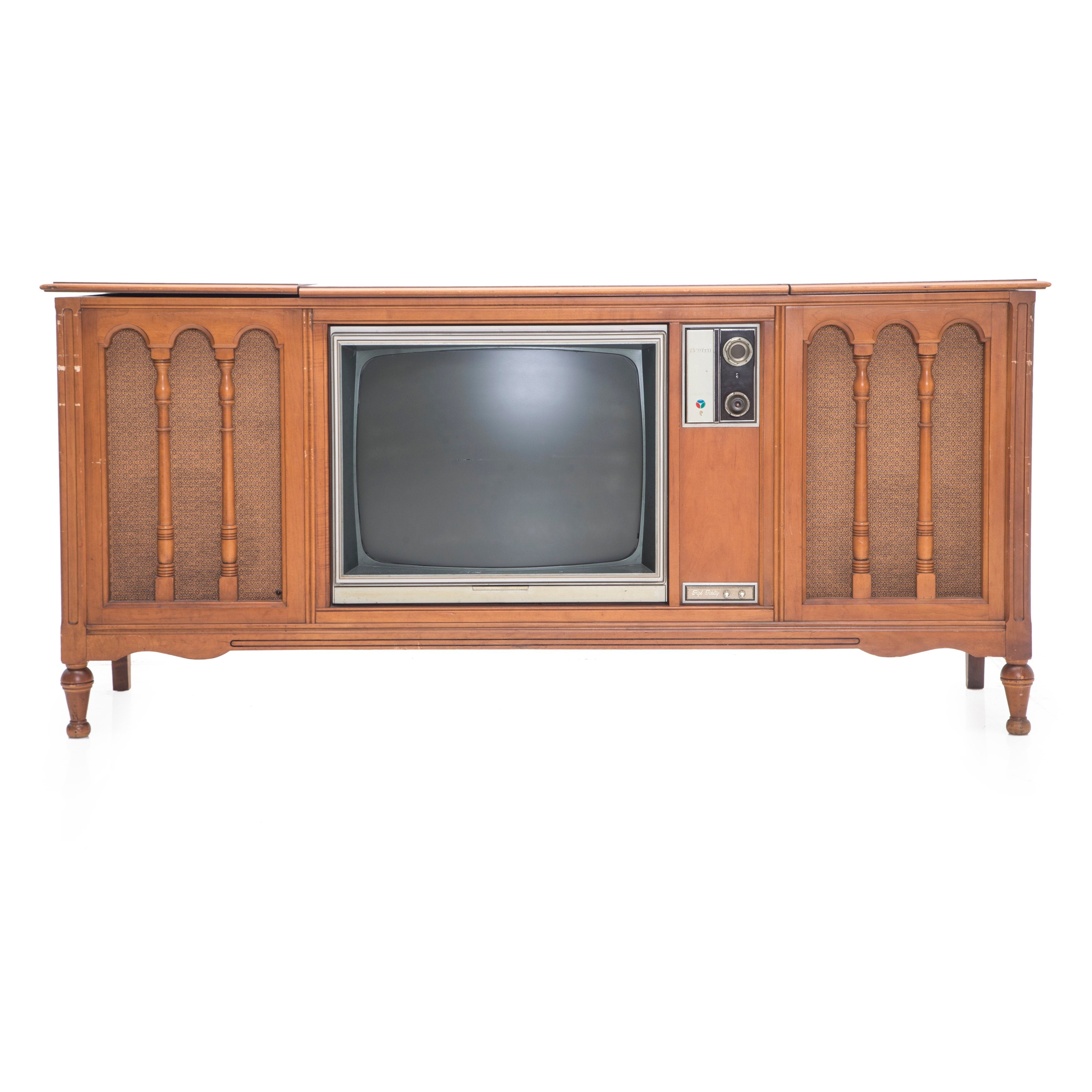The image showcases an antique console television, likely from the 1960s or 70s, displayed against a white background. The TV is embedded in a large, intricately designed piece of wooden furniture with a reddish medium brown finish. This console, which stands on four low legs, features several notable elements. The TV screen itself is framed in gray with a black screen, which has a slight shine at the top. Adjacent to the screen, there's a black and silver control panel featuring two dials. Flanking the screen are wooden-framed arch designs with mesh backgrounds that house the speakers. Above these sections, the console has three lids, with the left one slightly open, suggesting possible storage space. The sides of the console are decorated with carved column-like designs, adding to its vintage charm.